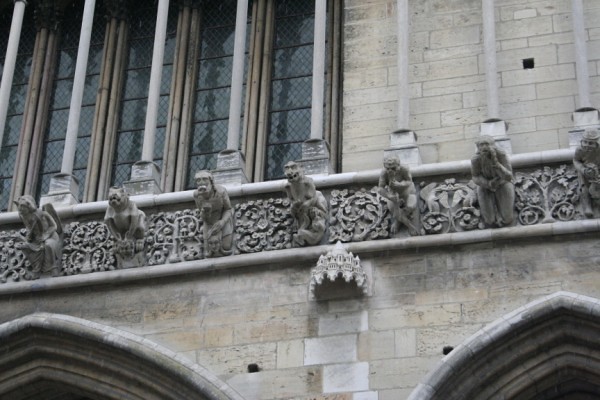This photograph, taken from the ground looking up, captures the intricate architecture of a gothic stone building, possibly a cathedral. The image prominently features the top sections of two archways at the bottom, suggesting entryways or tunnels. Above these arches is an ornate circular overhang, likely a light source at night. Adorning the building is an elaborate, carved frieze with botanical designs and curlicue letters, populated by seven unique winged gargoyles positioned in a line, angling from left to right. Higher up, slender columns frame tall, narrow leaded glass windows, which may look out onto a narrow walkway or balcony. The building showcases a color palette of light gray, white, and dark gray stones, with some stones appearing replaced, adding white contrasts to the otherwise gray structure.